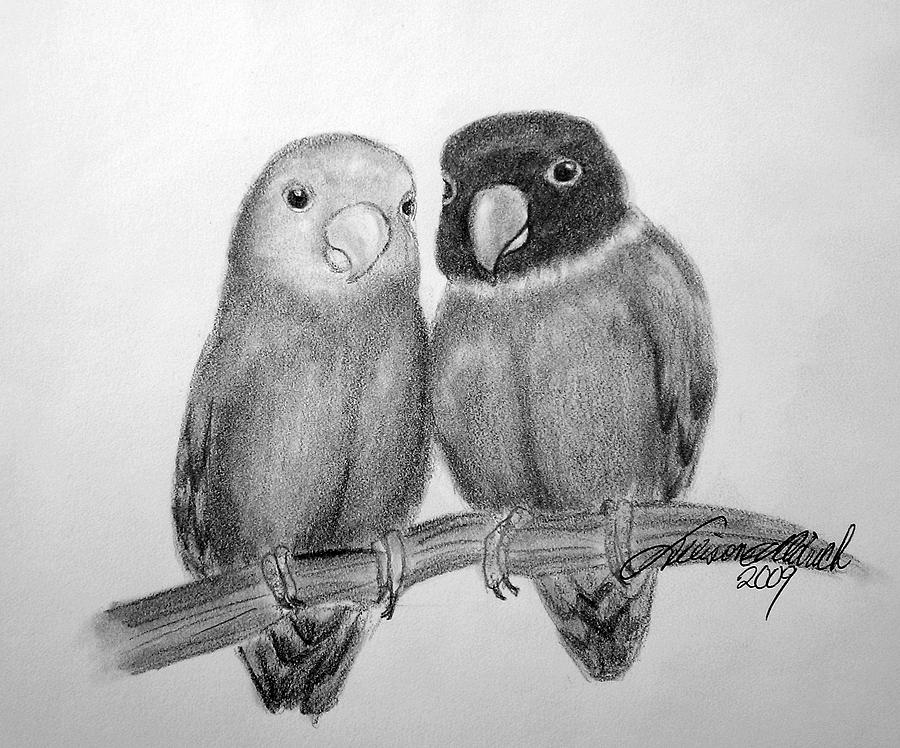This horizontal-rectangular pencil drawing, created in 2009 and signed by the artist at the bottom right, features two intricately detailed parrots perched side-by-side on a curved, textured branch. The bird on the left, slightly smaller and slimmer, has a lighter gray head and a softly smudged, layered appearance to its wings. Its face is lighter, with black eyes and a curved beak. The bird on the right stands out with its dark head and distinct white ring around its neck. It has a similarly curved beak and folded wings, and appears a bit more robust. Both parrots' feet clasp the branch securely, displaying the natural texture of the wood through delicate linework. The overall effect of the hand-drawn, black-and-white image is both detailed and evocative, capturing a serene moment between the two birds.